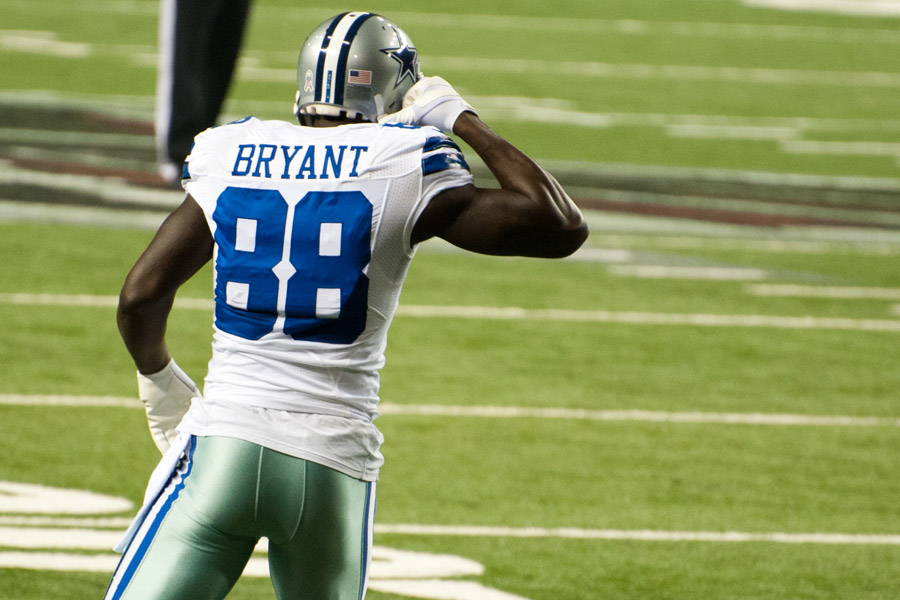The image depicts a muscular Black football player from the Dallas Cowboys standing on a green football field. The player's back is turned towards the camera. He is wearing a white jersey with navy blue lettering that spells "BRYANT" and the number 88. His pants are silver with blue and white stripes on the sides. He sports a silver helmet with a blue star and a blue central stripe. The player is wearing white gloves; one arm hangs by his side while the other is lifted, possibly adjusting his helmet. In the background, the green field has white stripes, and there's a person only partly visible, evident by their black pants with a white stripe.